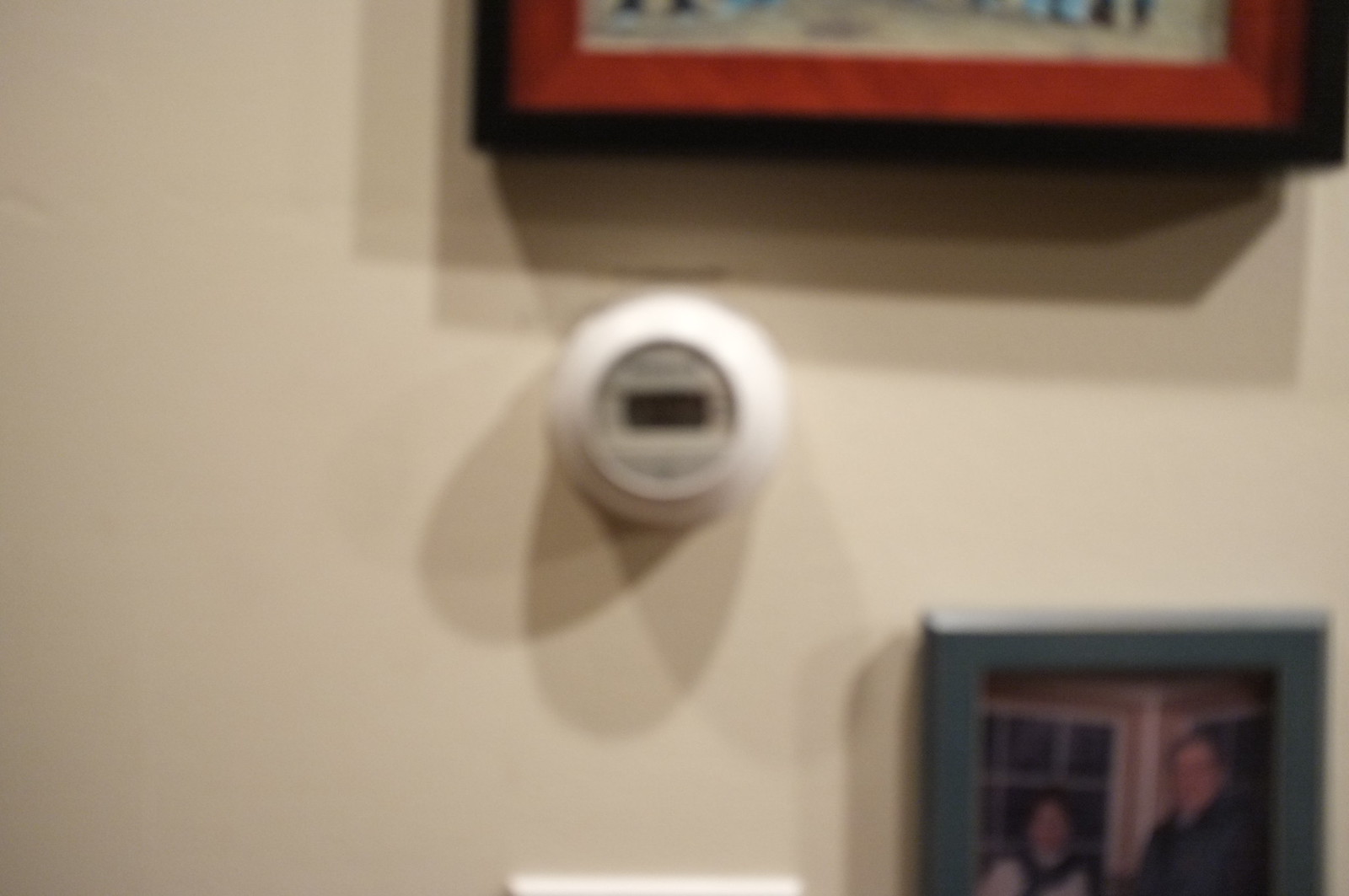A detailed photo reveals a beige wall adorned with several distinct elements. Central to the image is a round, white thermostat control that protrudes slightly from the wall. This device features a central circular display, possibly showing a tiny screen, and appears to have some writing positioned above or below it.

Above the thermostat, there's a framed picture with a dark brown or black frame and a red mat. Although the exact design of the picture is unclear, glimpses of beige and other colors are visible within the frame.

To the bottom right of the image, another framed photograph catches the eye. This black frame encases an image of a man and woman standing in front of windows. The man, possibly sporting dark hair and glasses, wears a dark suit. The woman has dark hair and dons a beige top with a dark brown collar. Both figures are shown from the waist up, and the background includes visible window panes with white trims, contrasting against the dark panes of the window.

Additionally, a small portion of a white electrical outlet is visible on the wall near the photograph of the couple. Each item displayed on the wall casts a shadow against the beige backdrop, contributing to the overall depth and detail of the scene.